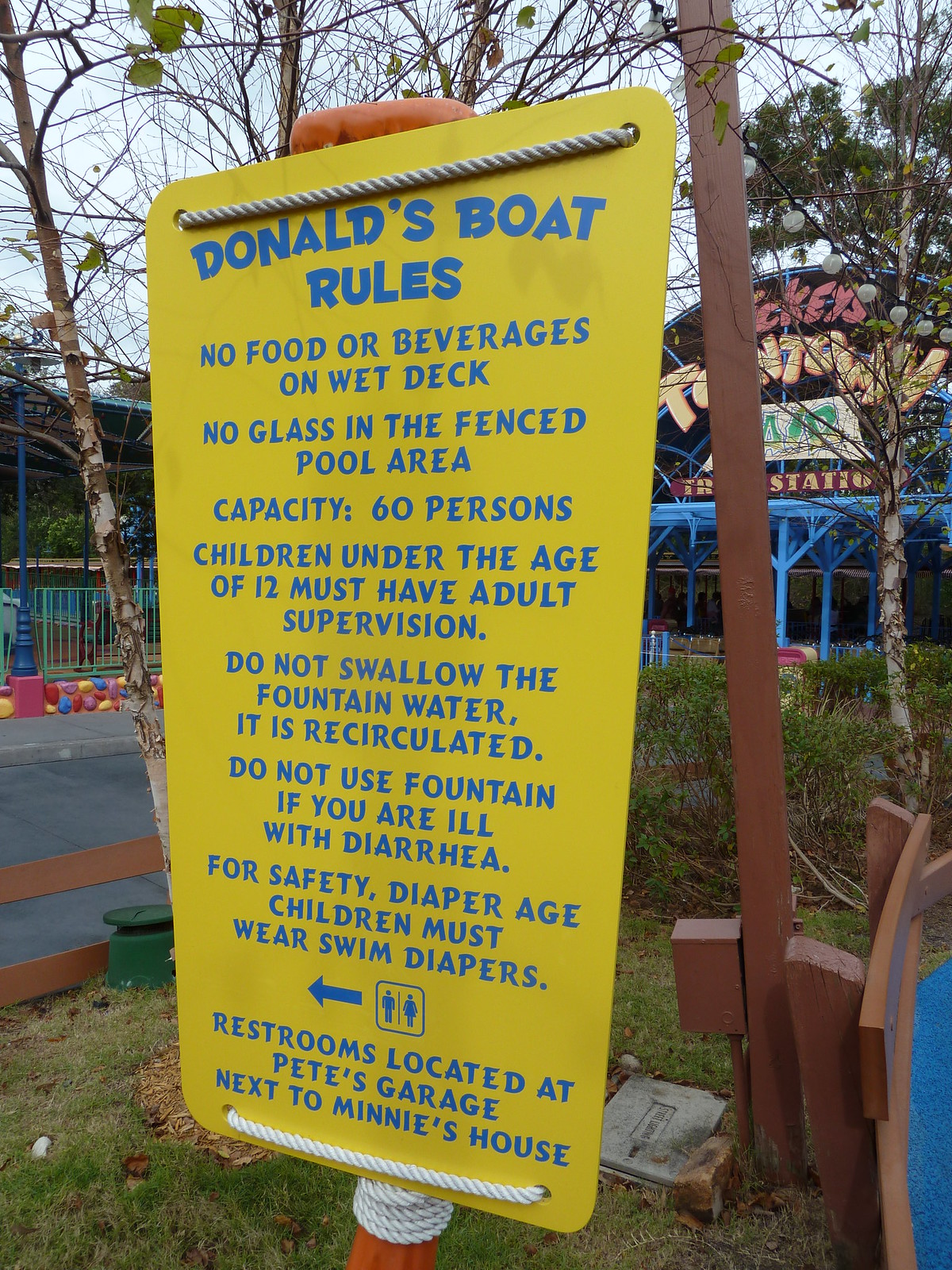The photograph captures a bright yellow sign prominently displayed in an amusement park, specifically in what appears to be the Disney-themed area of Mickey's Toontown. The sign, which is illustrated and tied to a pole with maritime-style rope, details the rules for a kiddie ride called Donald's Boat. The blue text on the yellow background states several safety instructions: no food or beverages on the wet deck, no glass in the fenced pool area, a maximum capacity of 60 persons, and requirements for adult supervision for children under 12. Additional safety warnings include directives not to swallow the recirculated fountain water, to avoid using the fountain if ill with diarrhea, and for diaper-aged children to wear swim diapers. To the left of the sign, there's an arrow pointing towards nearby restrooms located at Pete's Garage, next to Minnie's house. The background reveals some park buildings partially obscured by trees, with a possible sign reading "Mickey's Toontown." The photo, taken during the daytime, shows a somewhat moody atmosphere with sparse foliage on the trees and minimal human activity, adding to the serene yet slightly deserted ambiance.